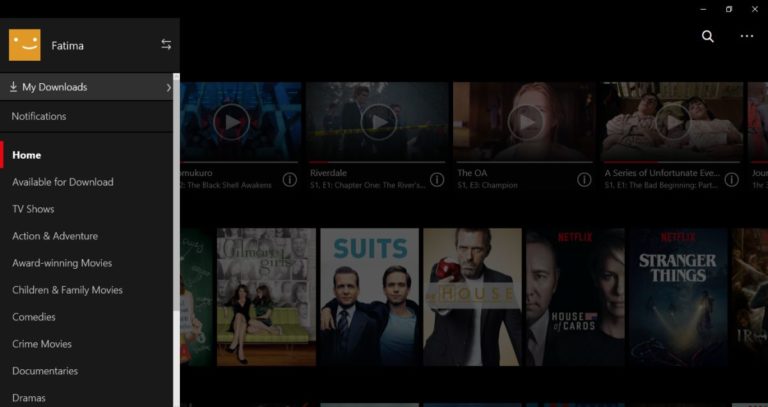The landscape image appears in a wide, rectangular format, reminiscent of a desktop monitor but almost twice as wide as it is high. The background is predominantly black and has no border, designed for a webpage named 'Fatima.'

**Header Area:**
At the top left corner of the header, there is an icon representing the Fatima logo. This logo consists of an orangish-brown square featuring two white dots near the upper corners, which resemble eyes, and a slightly off-center curve below the right dot that looks like a smile. Next to the logo, in white text, 'Fatima' is written. Further to the right, approximately a quarter of the way across the header, there are two vertically stacked arrows, with the top one pointing left and the bottom one pointing right. In the far right corner, there is a search icon - a white magnifying glass, followed by an icon of three horizontal dots indicating additional options.

**Left Panel:**
Taking up roughly 25-30% of the image width, the left panel has a background that transitions through various shades of gray. Right below the Fatima logo, there is a section labeled 'My Downloads' with a down-arrow icon beside the text and a rightward facing arrowhead on the far right. Below this, on a darker gray background, is the 'Notifications' section. The 'Home' section, highlighted with a thick red vertical line signifying it as the active section, has a black background and bold white text. Below 'Home,' there are nine more sections listed in white text (not bold), left-aligned: 'Available for Download,' 'TV Shows,' 'Action & Adventure,' 'Award-Winning Movies,' 'Children & Family Movies,' 'Comedies,' 'Crime Movies,' 'Documentaries,' 'Dramas.' Additional sections presumably extend below but are cut off in the image, indicating the presence of a scroll bar along the right side of this panel.

**Main Content Area:**
The remaining space to the right of the vertical white line (likely a scroll bar) is dedicated to movie content. The top half features two rows of video-related images. The top row consists of four screenshots with a white play button icon in the center, and underneath each screenshot is the title of the movie, a brief description, and a white circle icon with an 'i,' implying more information is available. The images are indistinct, but the leftmost image has a blue background, the second is gray, the third depicts a woman facing the camera, and the fourth shows two people lying in bed.

**Bottom Section:**
Below these screenshots, vertical portrait-style images, likely depicting DVD covers or movie posters, span the width. Five complete images are visible, with a sixth partially visible on each side. The second image clearly reads 'SUITS' in light blue uppercase text, showcasing two male actors. The third image features the TV show 'HOUSE,' with the lead actor Hugh Laurie depicted from the waist up, wearing a suit jacket, and 'HOUSE' is written in yellow font. The fourth image is from 'HOUSE OF CARDS,' displaying the actors Kevin Spacey and another character, with the title written in white. The fifth image is from 'STRANGER THINGS' with the title in bold, white, uppercase text at the top.

This composition of elements on the webpage offers an organized layout for a user interface focused on browsing video content, complete with navigation, search, and informational sections.